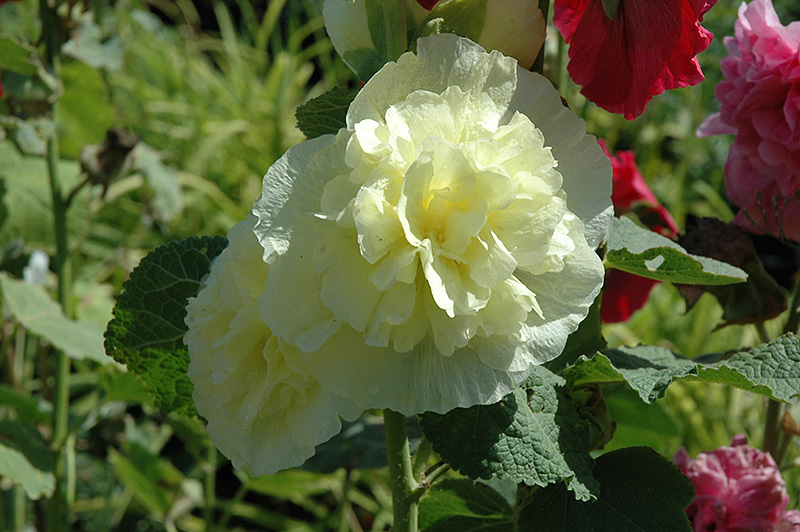The photograph prominently features a large, bright yellow-petaled flower positioned at the center, drawing immediate attention. This striking flower, with its broad petals fully spread out, is supported by a thick green stem accented with wide, dark green leaves, some of which show signs of being chewed. Surrounding the central flower are several other similar flowers in different colors—two with red petals and three with pink petals—crafted with similar petal designs and also growing on substantial green stems. In the blurry background, you can make out tall, thin blades of grass and a variety of lush greenery, adding to the natural setting. On the left side, a distinctive plant with a thick green stem is notable for its black bulbs on three of its branches, contrasting against the surrounding flora. The overall scene appears to be a vibrant, diverse garden or an undisturbed wild area, rich with different hues including various greens, reds, pinks, whites, and hints of black, adding depth and texture to the natural tableau.